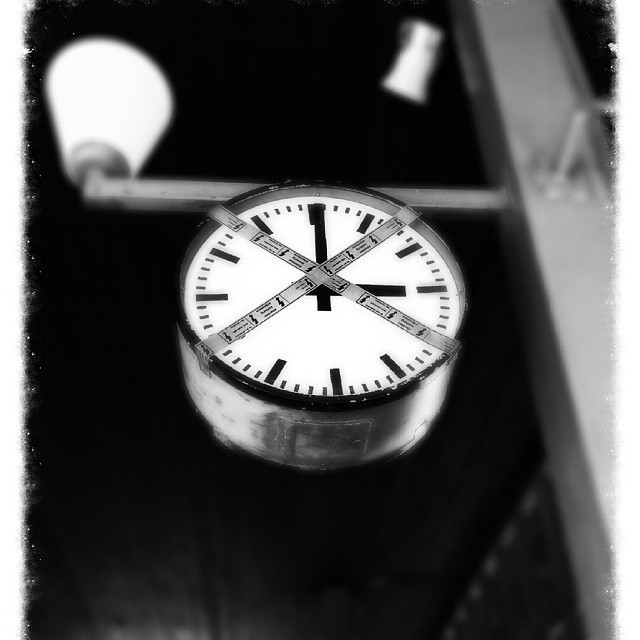The image is a striking black and white rendering that centers on a detailed timer or gauge. The timer dominates the picture, with its sharp focus contrasting against the blurred surroundings. Illuminated by directed lighting, the white dial of the gauge stands out, marked by rectangular indicators at what would typically be the hour positions and shorter minute markers in between. The hands of the clock are positioned precisely at three o'clock.

Prominently, strips of what appear to be tape or banding, adorned with black numbers or markings, intersect right at the dial's midpoint, where the clock hands converge. This adds an intriguing texture to the otherwise clean face of the gauge. The device itself is three-dimensional, with a black-banded edge framing the face, leading into a metallic body partially visible below. A distinct reflected shadow can be discerned at the area corresponding to six o'clock on a watch face.

This timer floats against a dark background, which reveals subtle hints of metallic paneling. Above the timepiece, a metal bar topped with a yellow cone-shaped element flares outward. This bar is affixed to a thicker metal strut on its right. Additionally, a ladder is faintly observable in the bottom left or right corner of the image, adding depth and context. Apart from the meticulously detailed timer or gauge face, the rest of the photograph remains intentionally out of focus, drawing the viewer’s attention irresistibly to the instrument at the center.